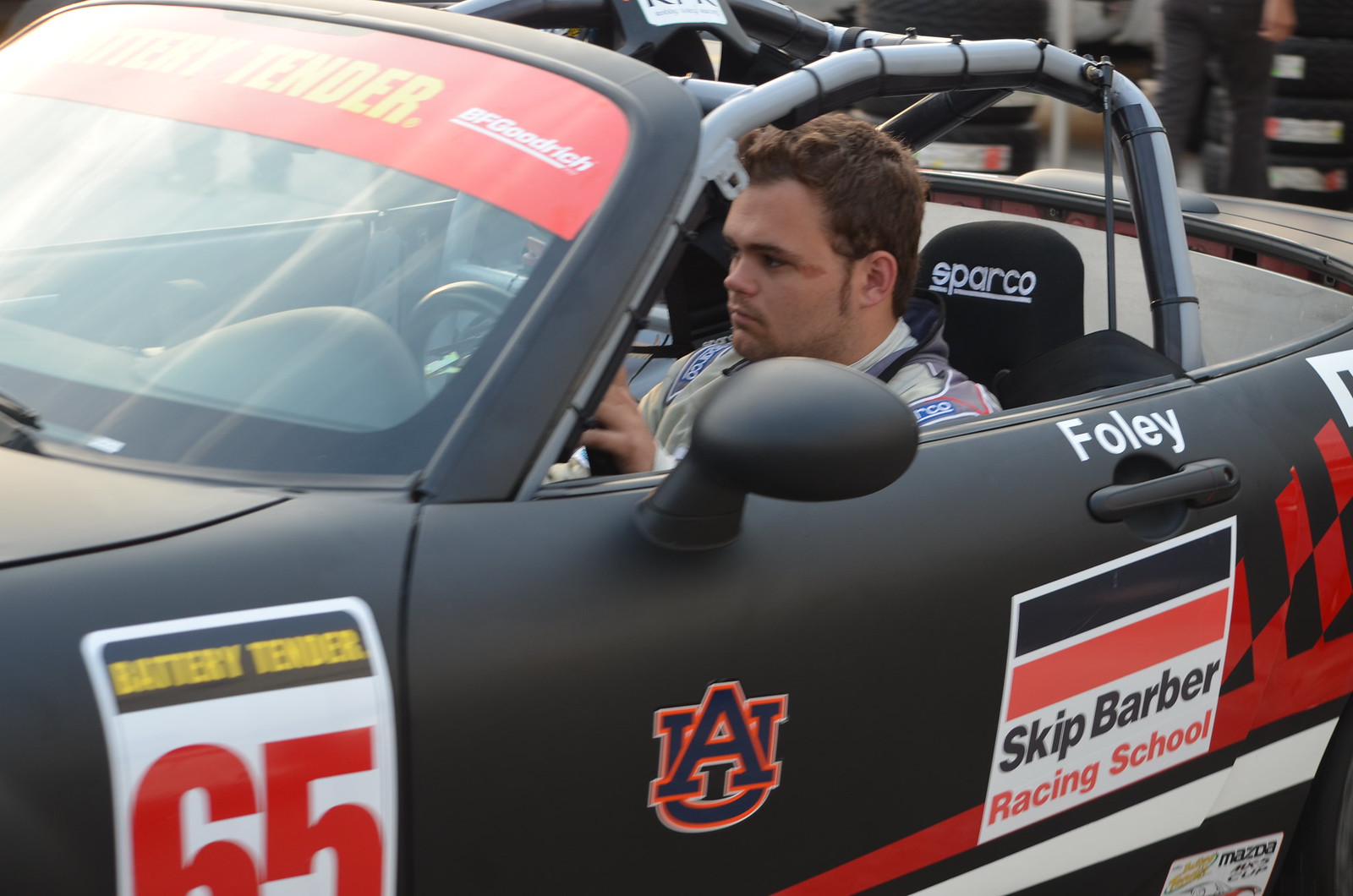An outdoor daytime image captures a young man with short brown hair and dark stubble, sitting inside a matte black convertible race car equipped with a crash cage and roll bars. He has a blank expression and holds the steering wheel, looking forward through the windshield. The car prominently features sponsorships: "Battery Tender" in yellow font and the number "65" in a black rectangle on the front. Nearby, there’s a University of Alabama logo, a black and orange flag symbol, and the text "Skip Barber Racing School," with "Racing School" in orange. Above the driver’s side door handle, the name "Foley" is visible in white letters. The background is blurred, suggesting a racetrack or racing event, with some obscured figures that appear to form a crowd, emphasizing the context of a racing school. The roll bars are clearly visible where the door frame should be and directly over the driver’s head. Additionally, the headrest bears the brand name "Sparco" in white letters.